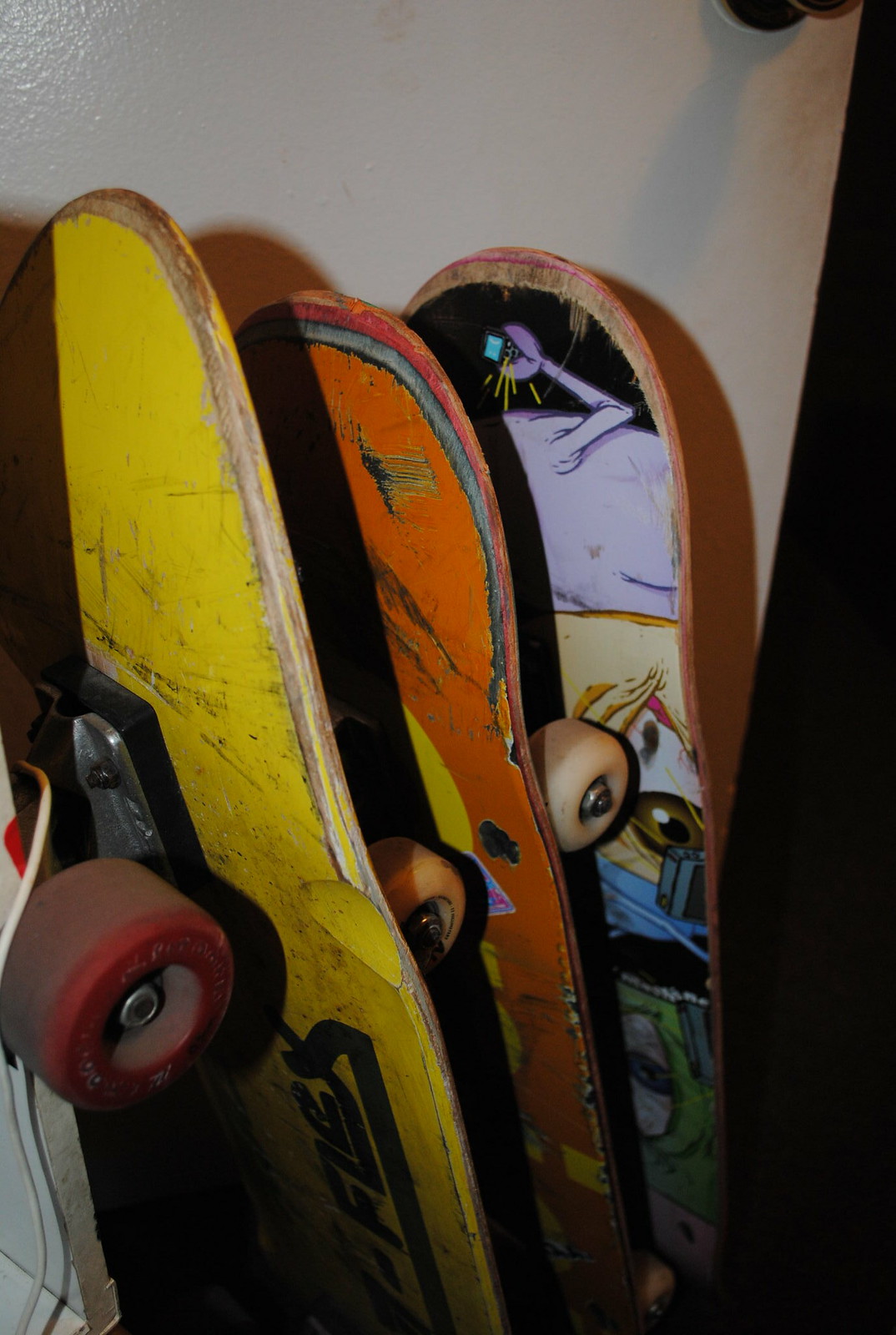This detailed photo features three well-used skateboards, standing upright and slightly angled to reveal both their sides and bottoms, leaning against a slightly ajar glossy white door with just the bottom of the doorknob visible in the top right corner. A dark shirt or fabric overlaps the door's top section. 

- The first skateboard on the left, visible from just above the red wheels, has a dirty yellow bottom with worn edges and black lettering partially legible as "flex."
- The middle skateboard, slightly shorter by a few inches, displays a vibrant orange bottom with matching wheels, featuring a mix of orange, pink, and blue graphics.
- The third skateboard, partially obscured, exhibits a more complex and artistic design: purple at the top, a central eyeball graphic, and the bottom transitioning to green, possibly depicting a hand.

The area is illuminated by artificial light, casting the skateboards into clear focus against the open door to a dark room. All three boards show signs of heavy use, with scuffs, dirt marks, and visible wood beneath the faded paint.